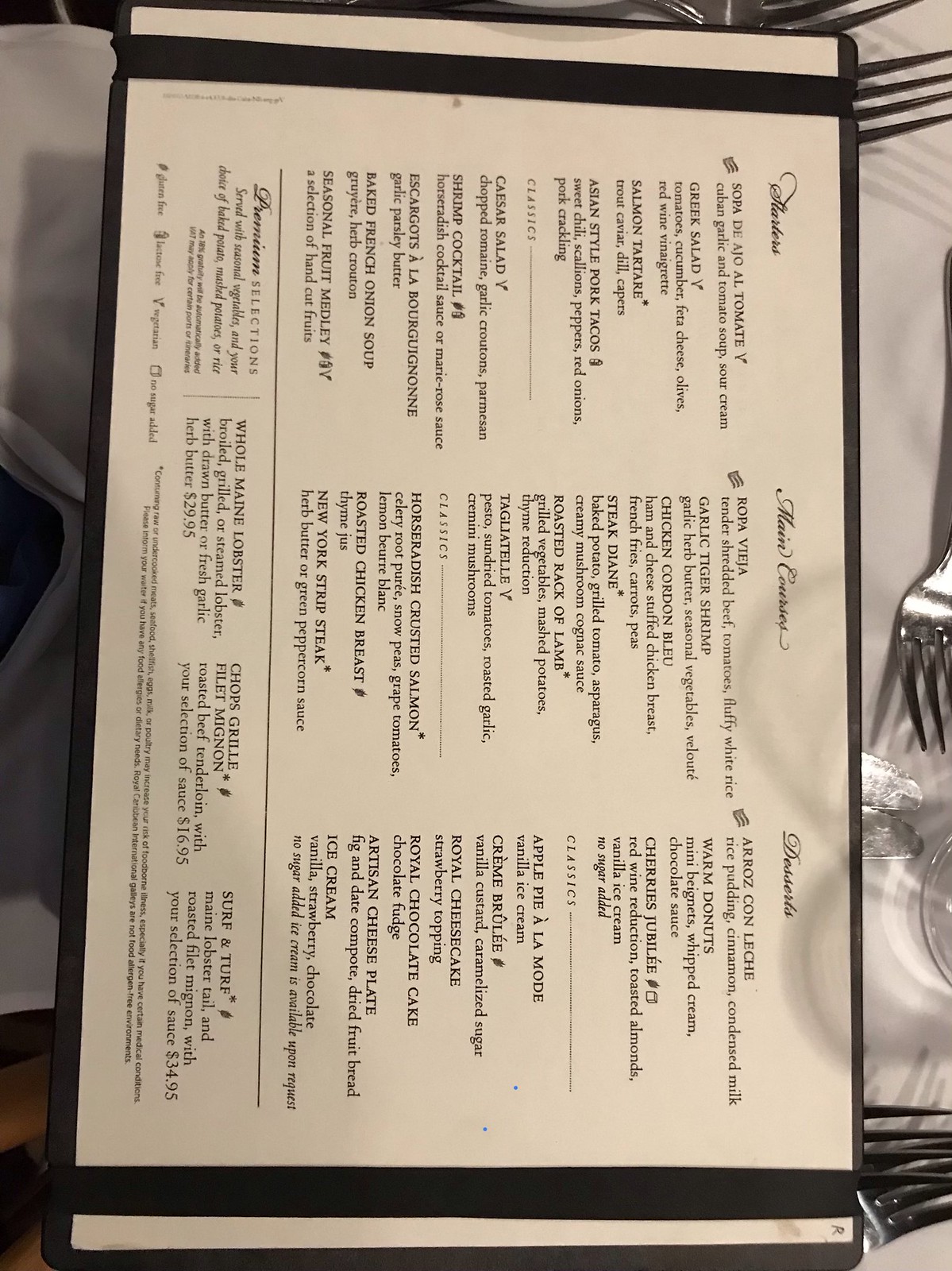A detailed photograph captures an elegantly arranged menu, presented in a unique manner. The menu, predominantly white with distinct black text, is initially seen in a landscape orientation. However, the photograph presents it upright, necessitating a tilt to the left for proper reading. The menu rests upon a pristine white linen tablecloth, adding a classic touch to the setting. Several pieces of cutlery surround the menu, subtly peeking from underneath, including two forks and two knives at the bottom right-hand corner, another fork alongside the right edge, and two more forks towards the top.

The menu appears to be of Greek cuisine, featuring items like Greek salad. Sections are neatly organized with italicized headers for Starters, Main Course, and Desserts. Each dish is listed with symbols indicating dietary preferences such as vegan or vegetarian options, and possibly a note if the item is served hot. Notably, desserts are positioned unusually at the top, followed by Classics and main courses in the center, with additional Classics and desserts listed below. At the very bottom, a legend explains the symbols used throughout the menu, ensuring clarity and ease for diners.